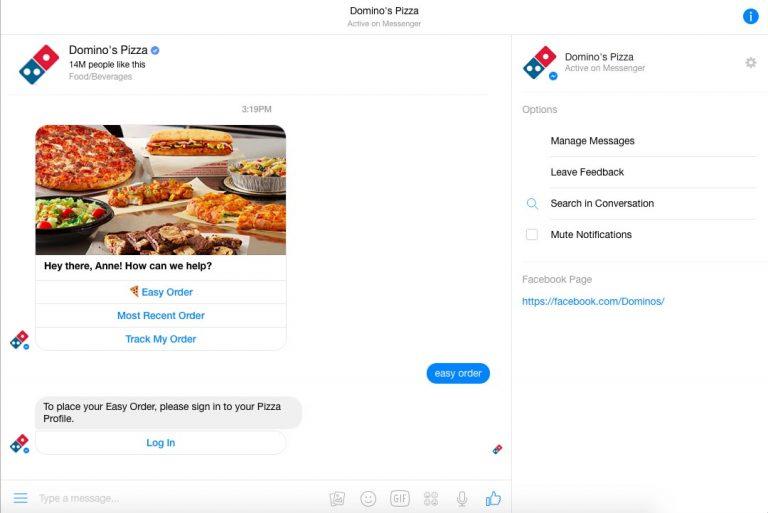**Detailed Caption:**

The image is a screenshot illustrating an interaction on the Messenger app, identifiable by its signature white background and user interface. At the top center, a small gray font indicates the status "Active on Messenger." Positioned just below this status, the profile name "Domino's Pizza" appears, suggesting that the user is engaged in a conversation with the Domino's Pizza official account.

On the left side of the screenshot, there is a larger section displaying a receipt of previous messages. The conversation history shows the Domino's Pizza profile, marked with the company's logo and a blue verified checkmark, denoting authenticity. The page has an impressive following of 14 million likes. A timestamp at 3:19 indicates the time of the latest message sent by Domino's, which includes a link for a survey, accompanied by a friendly greeting, "Hey there Ann, how can we help?" The message also features a stock image showcasing an assortment of food items offered by Domino's.

Below this, bullet-pointed options prompt the user to select among "Easy Order," "Most Recent Order," or "Track My Order." The user opted for "Easy Order," to which Domino's responded with instructions to sign in to their pizza profile for placing an easy order. The message includes a clickable blue hyperlink guiding the user to the login page. At the bottom of this section, the input bar is visible, complete with options to add an emoji, GIF, microphone input, or a thumbs-up icon.

On the right side of the screenshot, a smaller section reaffirms the interaction is with Domino's Pizza by again displaying their profile picture and confirming the "Active on Messenger" status. This side also features a settings icon, providing various options such as managing messages, leaving feedback, searching through conversations, muting notifications, and a direct link to the Domino's Facebook page.

Overall, the screenshot effectively captures the structured and user-friendly nature of customer support interactions through the Messenger app with Domino's Pizza.